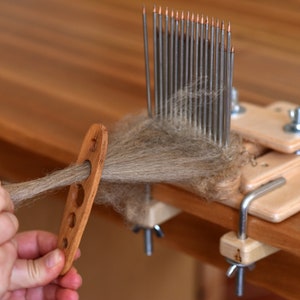In a woodworking shop, a photograph captures the scene on a brown wooden table with visible grain running from the top left to the bottom right. A silver structure, likely a wool spinner or other fiber processing tool, is firmly attached to the table. This tool features small pins and holes, used for threading yarn or wool fibers. The light beige, sandy gray fibrous material is being meticulously pulled through these holes by a pair of hands positioned in the bottom left corner. The left hand steadies the wooden tool, which has a dark mahogany and reddish-brown hue, while the right hand carefully pulls the fibers through. The setup and the process evoke a traditional craftsman atmosphere, with the interplay of varying shades of beige, gray, and brown creating a rich, detailed composition.